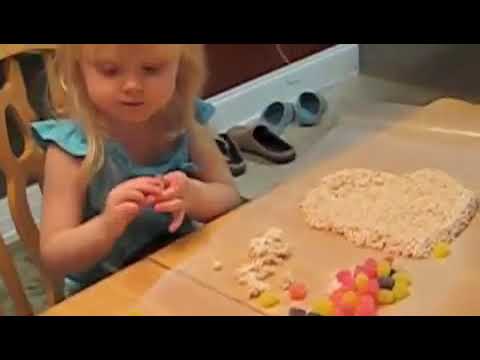This image shows a little blonde girl wearing a blue sleeveless top, sitting in a wooden chair at a light brown wooden table. She is focused on something in her hands, covering it with her fingers, so the item remains obscured. Spread out on the table in front of her is a piece of wax paper with what appears to be the beginnings of a Rice Krispie treat. To her right are multicolored gumdrops and possibly some other candy. The wooden table has a sectional design, indicated by a line running through it. In the background, a maroon wall with a white baseboard is visible. Additionally, there are pairs of blue and brown shoes lined up against the wall, resting on linoleum flooring with a section of carpet visible to the left. The image itself appears to be a still frame from a low-resolution, low-quality video.